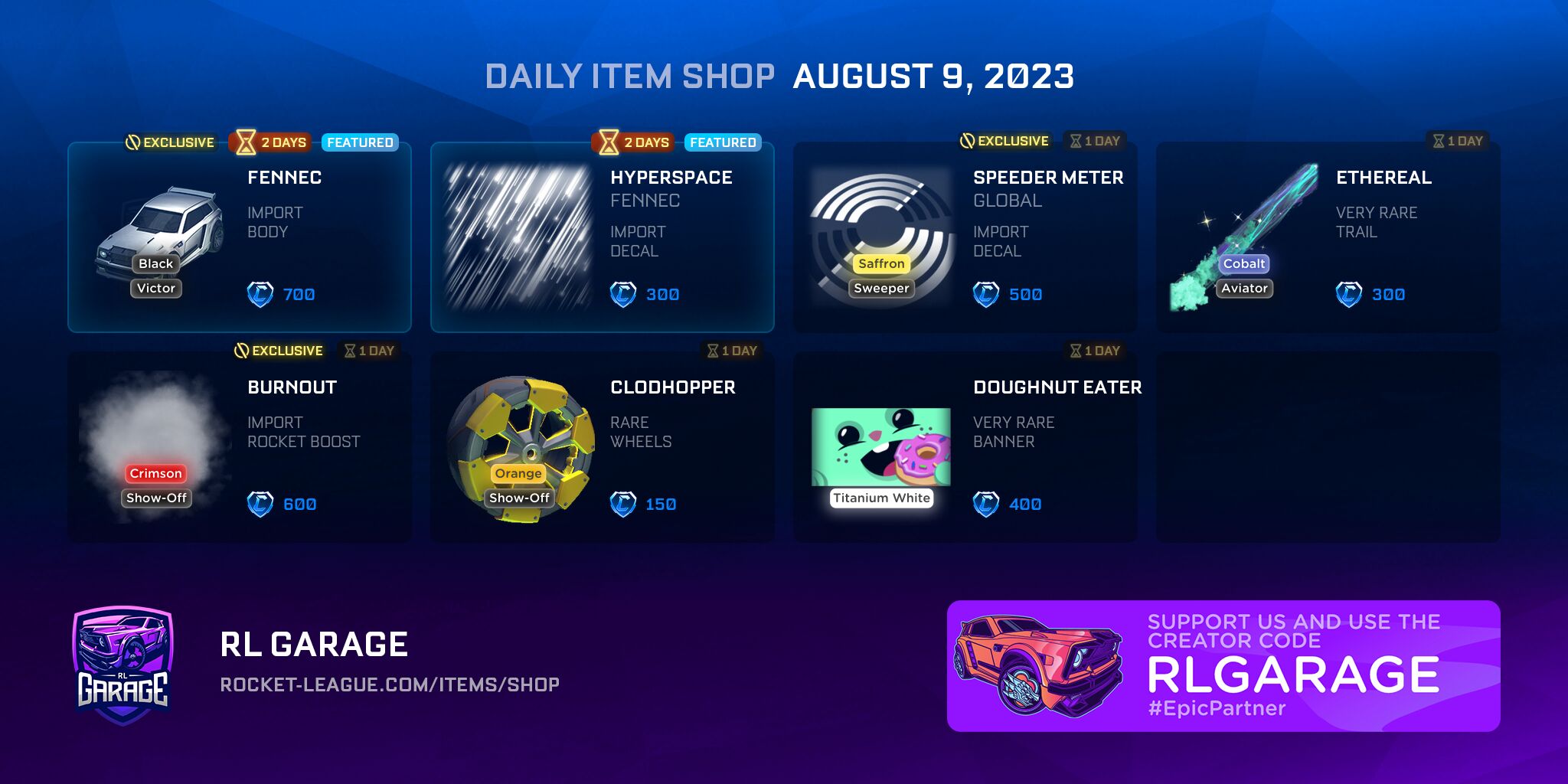This image depicts a game menu titled "Daily Item Shop - August 9, 2023." The background features a gradient transition, starting with a medium blue at the top, merging into a darker blue in the center, and finally transitioning to a purple hue at the bottom. The image is horizontally rectangular.

At the top of the image, bold block letters display the title. Below the title, there are eight rectangular sections resembling file folders, arranged in two rows of four. Each folder represents different car accessories or upgrades available for selection, including options like Fennec, Hyperspace, Speedometer, Ethereal, Burnout, Clawhopper, and Donut Eater.

In the bottom left corner, there is a purple badge logo that features an image of a car, accompanied by the text "Garage." Below the badge, a URL is displayed: "rlgaragerocketleague.com/item/shop." 

On the bottom right side, there is a lighter purple rectangle with an image of a car, along with the text: "Support us and use the creator code rlgarage #epicpartner."